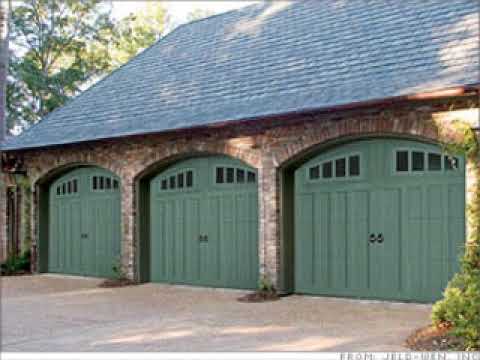The image is a square photograph with a distinct artistic style, heavily obscured by numerous horizontal lines that create a static-like effect, reminiscent of an old VHS tape. The lines, appearing as gray and white streaks, blend with the grayscale ambiance of the image, lending a filtered, almost blurred appearance. The image's borders are solid black on either side, framing the scene within. 

Amidst this visual distortion, a black convertible is either pulling into or backing out from what appears to be a large, elegant house. The vehicle contains two people, with the driver waving towards the house. The house itself features a prominent porch with white wooden pillars. On the right side of the image, there is a faint hint of a red door and possibly windows illuminated from within. The bottom portion of the image appears more gray, gradually merging with the obscuring lines that dominate the center. Despite the heavy obscuration, the photograph captures a moment imbued with a sense of mystery and nostalgia, heightened by its deliberate, stylized presentation.